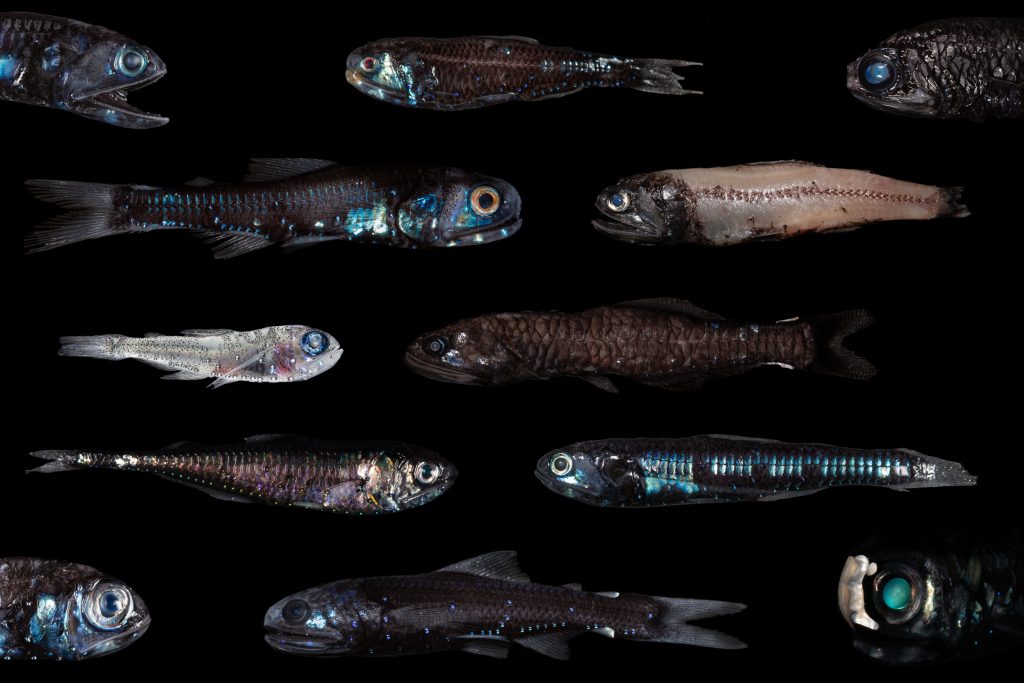The image showcases an array of surreal-looking fish set against an all-black background. These fish, appearing to be an artistic or digital assemblage rather than real specimens, are lined up in non-natural, horizontal rows—totaling five rows. The fish vary in color, predominately exhibiting dark shades of black, brown, and deep blue, with a few exceptions. Noteworthy among them is one fish in the upper right corner featuring an enormous blue eye, another in the bottom left flaunting a bulging blue eye, and a light-colored fish in the middle left. A peculiar fish in the center-left is white with a strikingly large blue eye, resembling an ancient or prehistoric species with exaggerated features like enormous eyes and rounded, toothless mouths. These whimsical creatures appear otherworldly or extinct, adding to the mysterious and haunting ambiance of the composition.